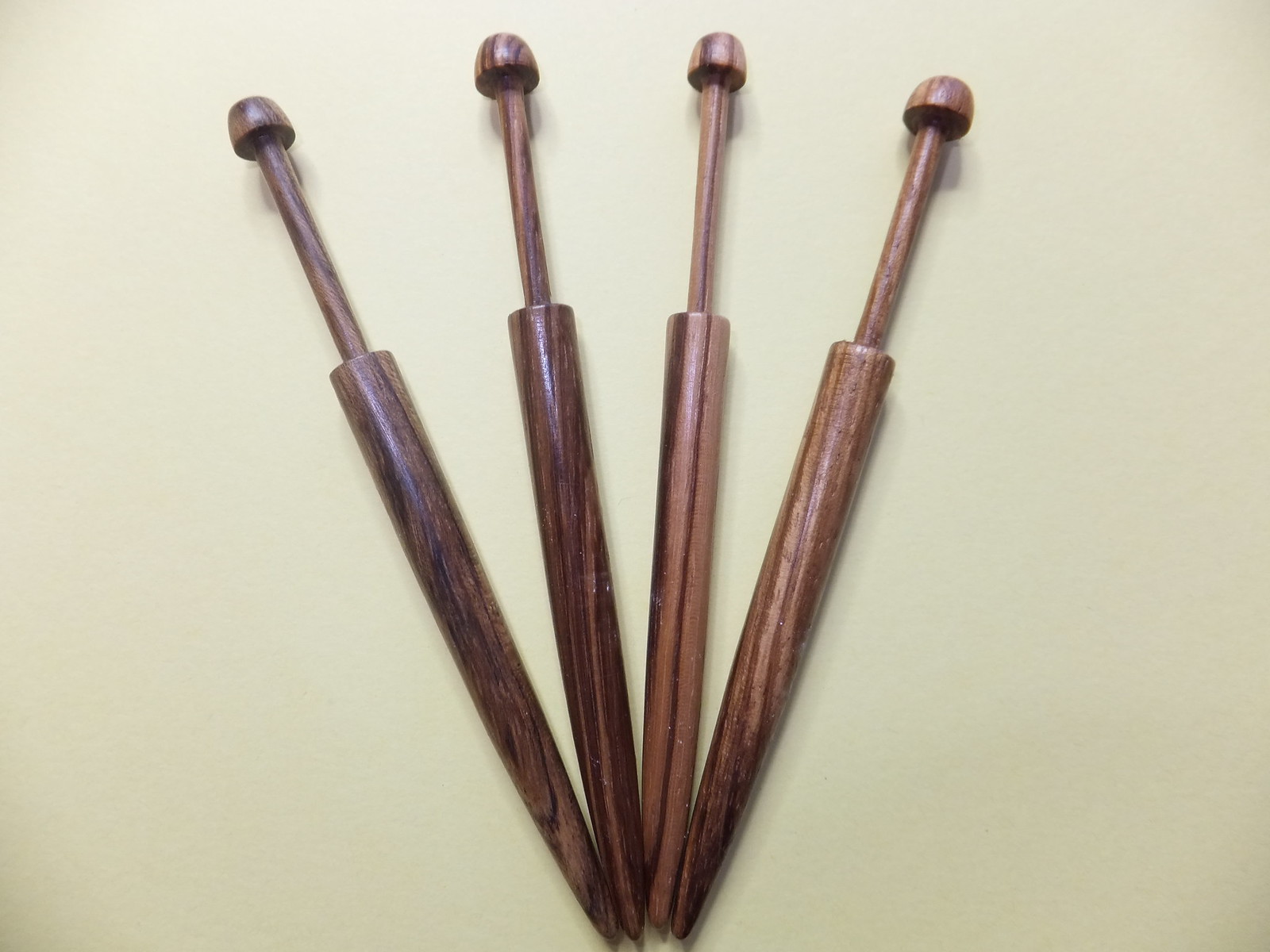This detailed close-up photo captures four finely finished wooden objects, reminiscent of pens or skewers, arranged in a fanned-out position on a plain cream background. Viewed from above, the objects vary in shades of brown—two darker and two lighter. The top portion of each object resembles that of a pen with a cylindrical body tapering to a rounded, polished tip, while the opposite end features an oval-shaped top, much like the push button of a pen that has yet to be pressed. The smooth, well-defined wood grain and glossy finish add an elegant touch, enhancing their visual appeal against the stark background. They appear slightly diagonal, with their tips jumbled closely together, gradually spreading out towards the top.